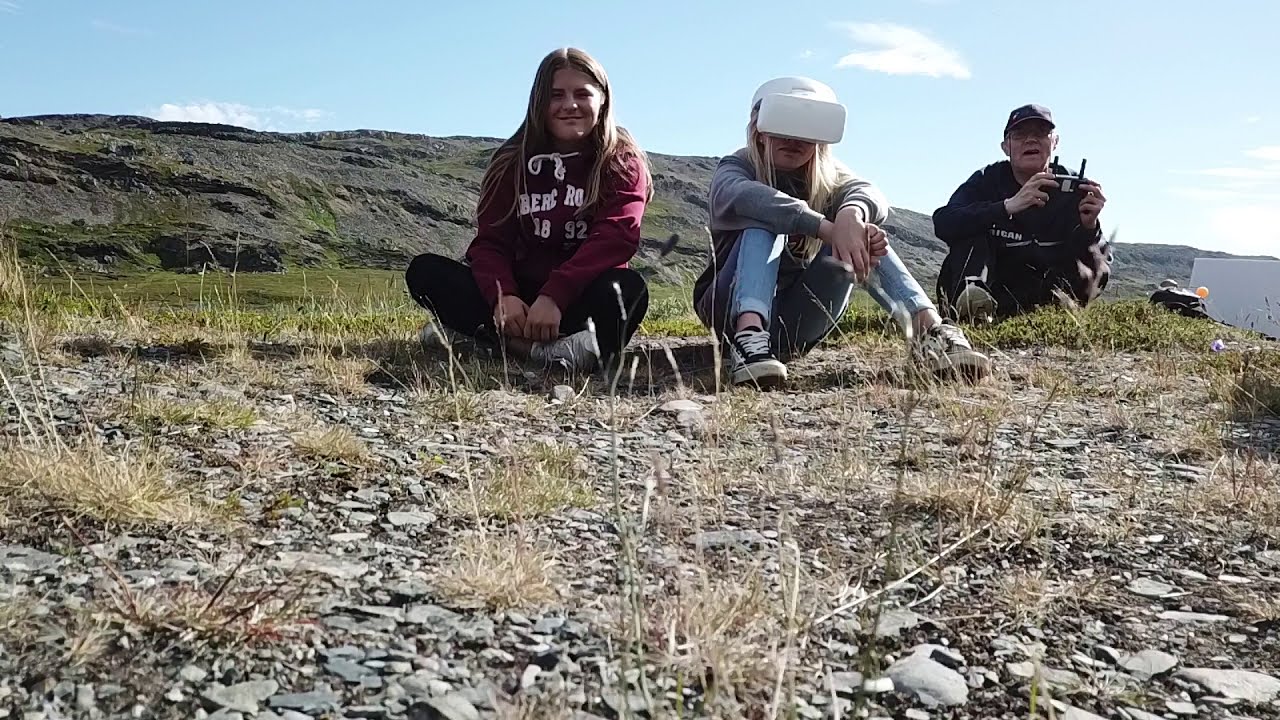Three individuals, likely a family, are seated on rocky, sparsely vegetated ground under a bright blue daytime sky with a few scattered white clouds. The scene shows two young girls, both of Caucasian descent, and an older man, possibly their father. The girl in the center has long light brown hair, parted in the middle, and is smiling at the camera. She is dressed in a red long-sleeved top with white pull strings and lettering, dark pants, and white shoes. To her right is another girl wearing a virtual reality headset, which covers her eyes. She has long blonde hair and is dressed in a gray sweatshirt, blue jeans, and black and white sneakers. The older man, positioned slightly behind them to the right, is holding a remote control, likely for a drone. He wears a black baseball cap, glasses, and dark-colored clothing. The backdrop features a green open plain extending towards rocky mountains in the distance, adding a natural charm to the setting.